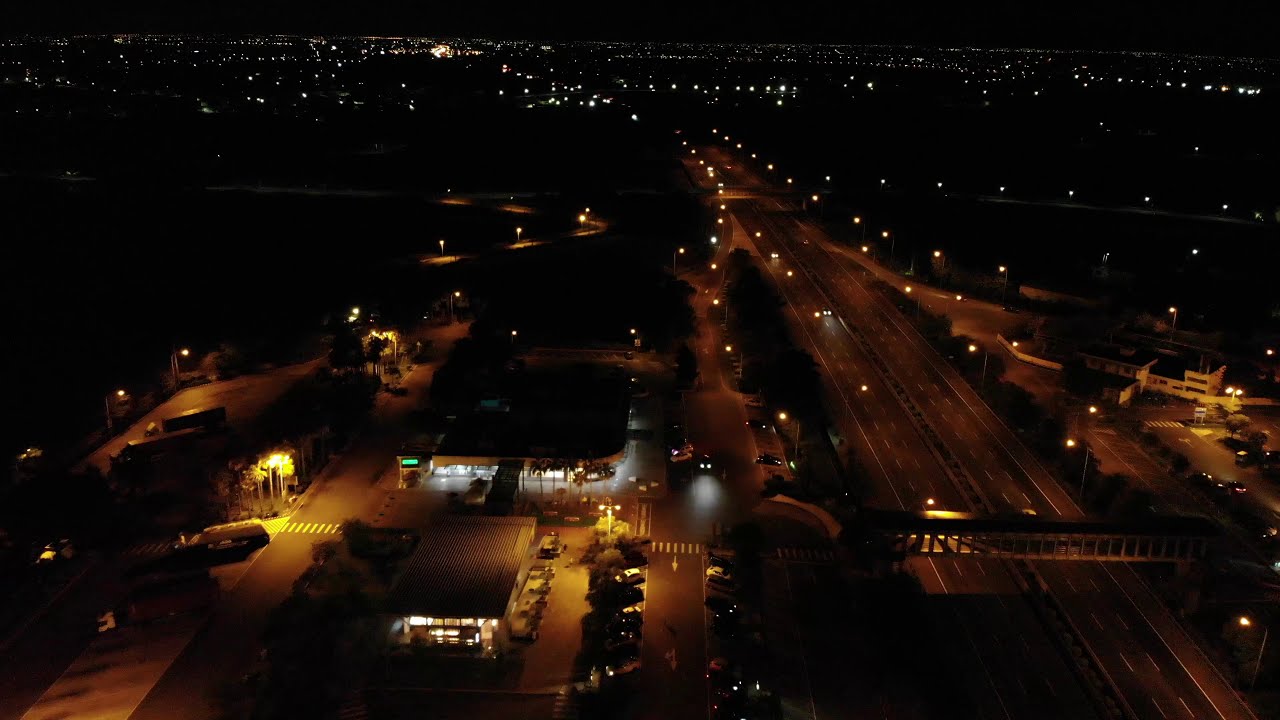This image is an aerial night view of a suburban area featuring a prominent, nearly vertical road running through the center, slightly veering left. The setting is primarily black due to the nighttime ambiance, punctuated by various lights. Bright white streetlights line the road, creating a stark contrast against the dark surroundings. Along the road, particularly towards the bottom of the image, several low-rise buildings are visible. On the left side, there are clusters of structures with adjacent street lamps and a few cars parked outside, likely in a parking lot or along the street. On the right side of the road, there's a single house standing out amidst the darkness. The foreground reveals more details, including a white crosswalk illuminated by the streetlights, highlighting the road’s path. As the scene stretches into the distance, it fades into a sea of darkness spotted with occasional lights, giving the impression of a quiet suburban night with minimal traffic.